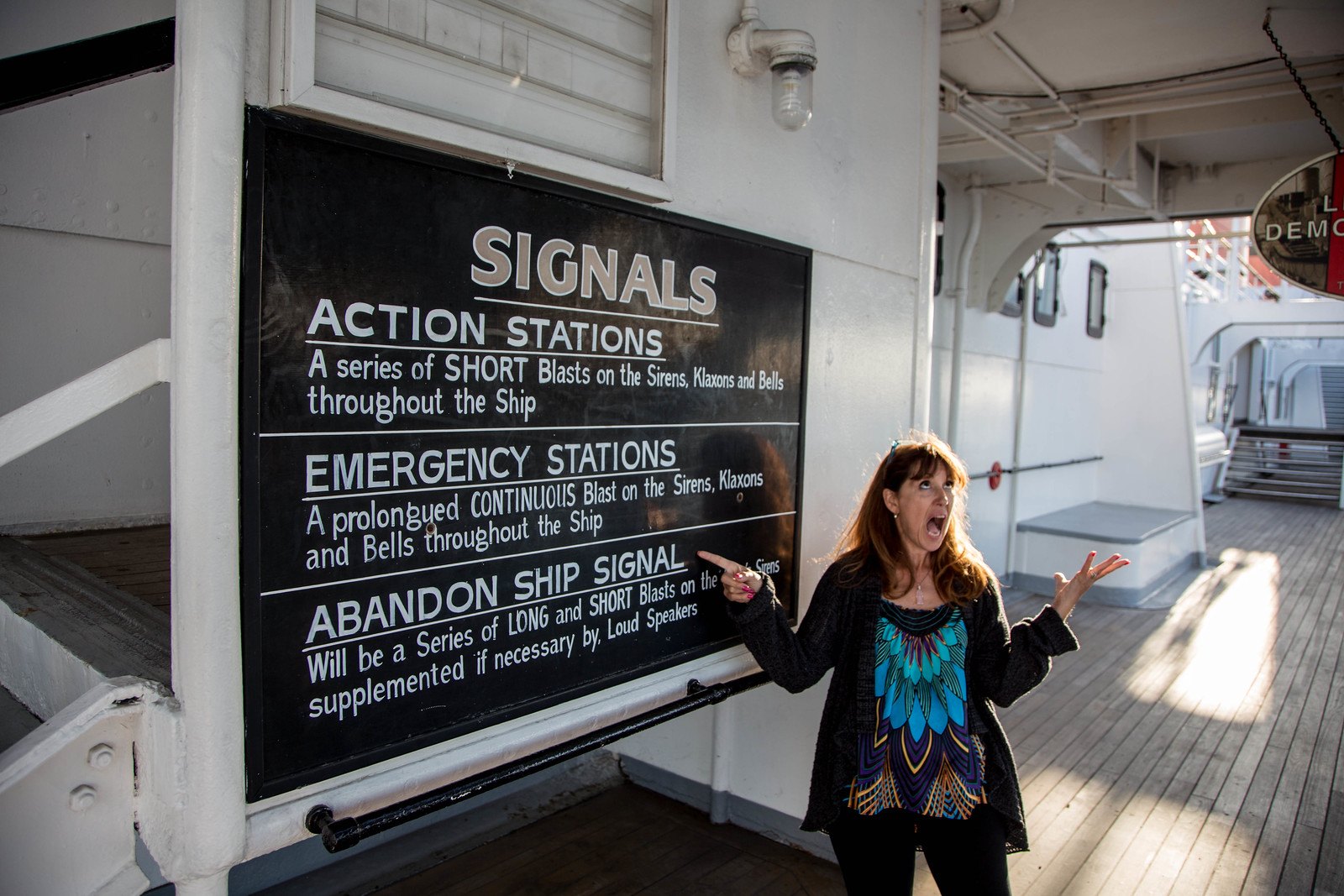The image depicts a woman standing outdoors, seemingly on a ferry or cruise ship, indicated by the visible white walls, metal structures, and wood board slats beneath her feet. She has reddish-brown hair cascading over her shoulders and is wearing a light-dark jacket over a floral shirt with blue and gold trim, along with dark pants. Her mouth is wide open as if she is yelling, and she has her hands outstretched, possibly pointing or signing for the deaf. She stands next to a blackboard with white lettering, which provides safety signals: "Action Stations" with a description of series of short blasts, "Emergency Stations" detailing a prolonged continuous blast, and "Abandoned Ship Signal" describing a series of long and short blasts. The blackboard is affixed to the wall near some installed lights and a pair of steps, and there are a couple of windows visible in the background. The overall setting hints at a maritime environment with safety instructions clearly displayed.